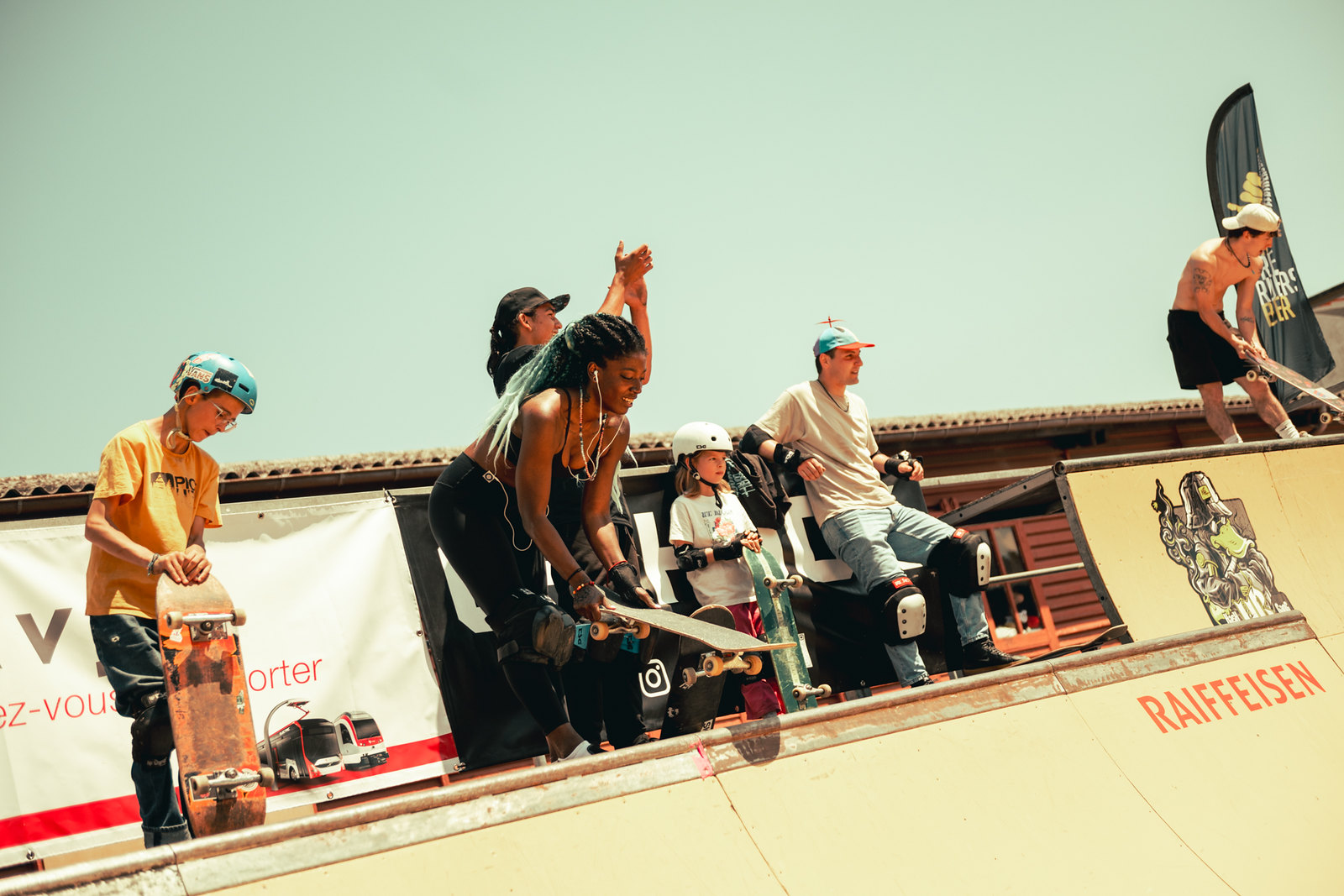In this outdoor photograph taken at a skateboarding competition, the scene is set against a hazy sky, tinted seafoam green. The image captures six skateboarders atop a half-pipe ramp bearing the sponsor's name "Raiffeisen" in red along with a sticker graphic. The diverse group includes a shirtless white man with tattoos on his shoulder and leg, wearing black shorts and a backwards white hat; a black woman with long braids featuring blue ends, dressed in a black tank top and black pants, holding her skateboard as she prepares to drop in; a young Caucasian boy in a yellow t-shirt with a blue helmet and orange-bottomed skateboard; a child, likely a girl, with long blonde hair, clad in pink pants, a white t-shirt, and protective gear including elbow pads, wrist pads, and a white helmet, holding a green skateboard; a Caucasian girl with knee pads and a white helmet, listening to earbuds, smiling as she positions her skateboard; and another man who stands in the background clapping, contributing to the supportive atmosphere. The details of attire, accessories, and actions highlight the participants' readiness and anticipation to ride the ramp.